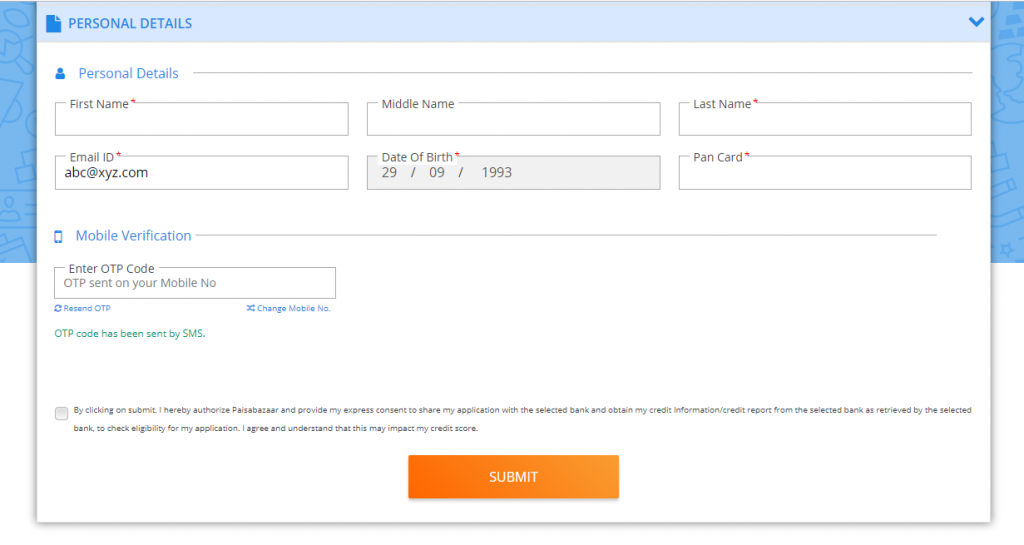Screenshot of a Form Interface for Personal Details Submission:

At the top of the form, a header labeled "Personal Details" is displayed, accompanied by a dropdown arrow that allows users to minimize or maximize the form. Below the header, an icon of a person is present, signifying the nature of the section.

The form fields are structured as follows: 
1. **First Name:** Marked with a red asterisk indicating it is a required field.
2. **Personal Name:** An optional field without a red asterisk.
3. **Last Name:** Another required field, also marked with a red asterisk.
4. **Email ID:** Contains the placeholder or predefined value "abc@xyz.com."
5. **Date of Birth:** A required field with the format "29-09-1993."
6. **PAN Card Number:** Also marked with a red asterisk, indicating it is mandatory.

Below the personal details section, there is a segment for mobile verification:
- The instruction to "Enter OTP Code" is displayed, noting that an OTP code has been sent to the user's mobile number.
- Options include a clickable "Resend" link and a "Change Your Mobile Number" link.
- A message confirms, "OTP code has been sent by SMS."

At the bottom of the form, there is a consent checkbox accompanied by a statement: "By clicking on submit, I hereby authorize [text partially visible] and provide my consent to share my application with the selected [text not fully legible]."

Finally, the form concludes with a prominent orange "Submit" button for submitting the completed details.